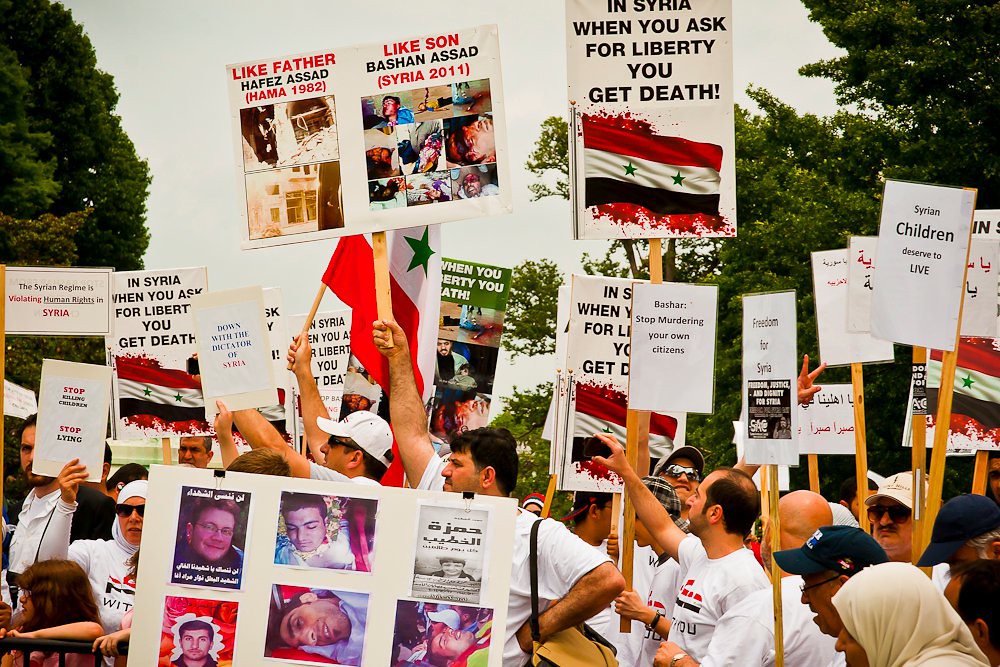This photograph captures an outdoor demonstration in a densely treed area, with overcast skies adding a somber tone. The scene features around 20 individuals, predominantly men, but with some women present, all clad uniformly in white t-shirts and long-sleeve shirts, each bearing a logo and slogan that is not completely discernible. They are standing quietly, not shouting, and holding up white poster boards mounted on brown wooden sticks. The posters are filled with powerful messages and graphic images, primarily focusing on the crisis in Syria. One prominent sign reads, "In Syria, when you ask for liberty, you get death," another states, "Syrian children deserve to live." There is a poignant comparison between the Assad regime, with one sign stating, "Like father, Hafez Assad, Hama, 1982," and "Like son, Bashar Assad, Syria, 2011," both accompanied by images of bloodied bodies and war destruction. The protest highlights the dire human rights situation in Syria, with numerous placards echoing the call for freedom and depicting the devastating impact on civilians.